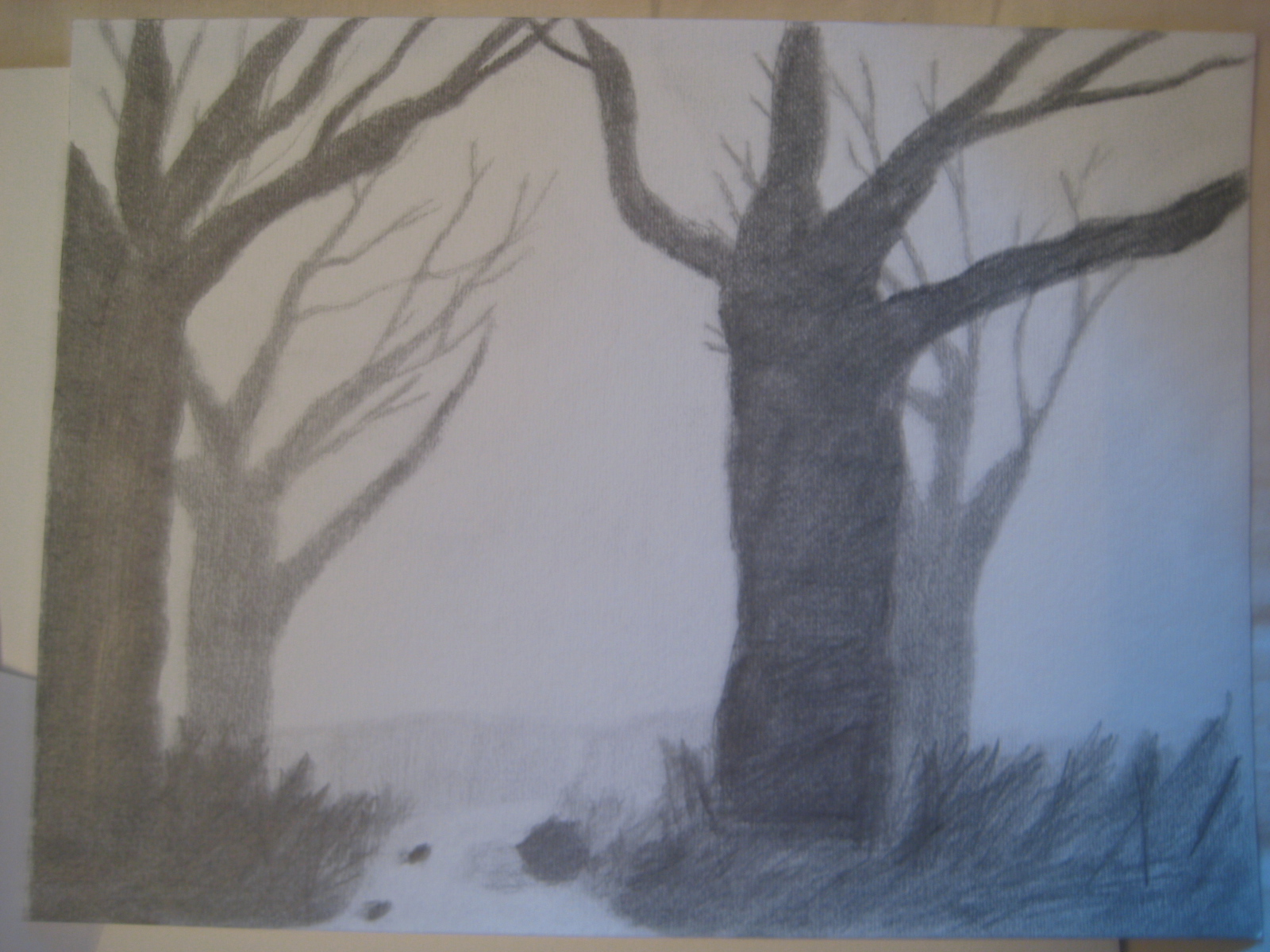This image is a detailed pencil sketch depicting a wintry forest scene. The tall trees, rendered in a dark, bold black, stand prominently against the stark white paper, their numerous bare branches reaching out in intricate patterns. The absence of leaves both on the trees and on the ground suggests a cold, snowy day, capturing the dormant state of nature in winter. 

In the foreground, sketchy tufts of grass peek through the snow, adding texture and depth to the scene. Nestled in the background, a wooden gate is subtly visible behind the trees, contributing to the quiet, serene atmosphere of the composition. The forest comprises four prominent trees, each with an elaborate network of branches, evoking a sense of stillness and solitude. The artist’s meticulous attention to detail in this monochromatic drawing creates a vivid portrayal of a tranquil winter landscape.